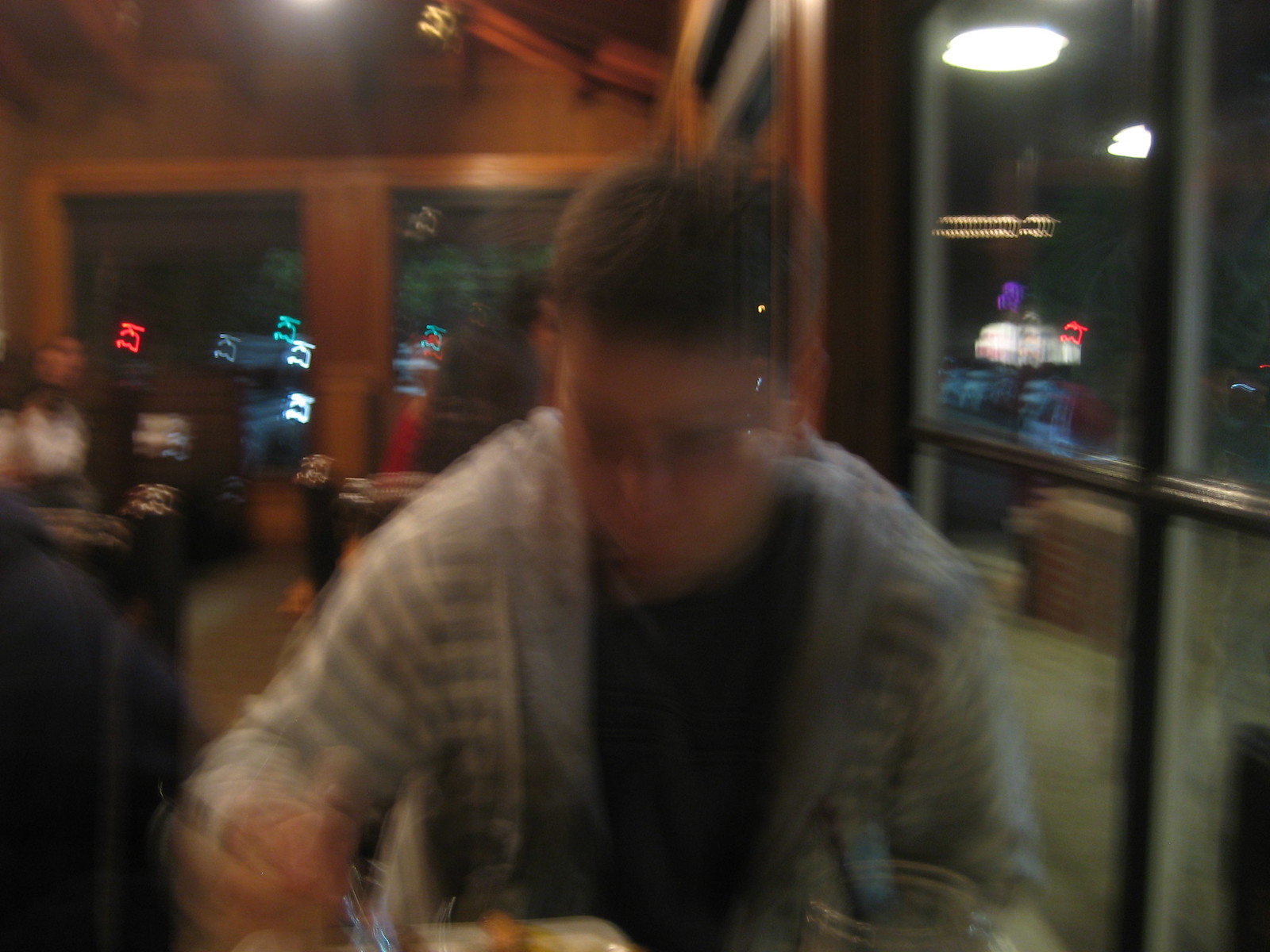In this candid, slightly blurry photograph, a man is captured at a modestly lit restaurant, engrossed in his meal. The setting appears to be a typical evening, evidenced by the darkened windows at the back and to the right of the room, illuminated by street lights outside. The man, wearing a light blue and white striped jumper over a black t-shirt, is focused on his food, his brownish hair slightly tousled. The background reveals the dim, cozy ambiance of the restaurant with wooden walls and doors. Other patrons are faintly visible, their forms blurred, adding to the intimate and unpretentious atmosphere of the scene.